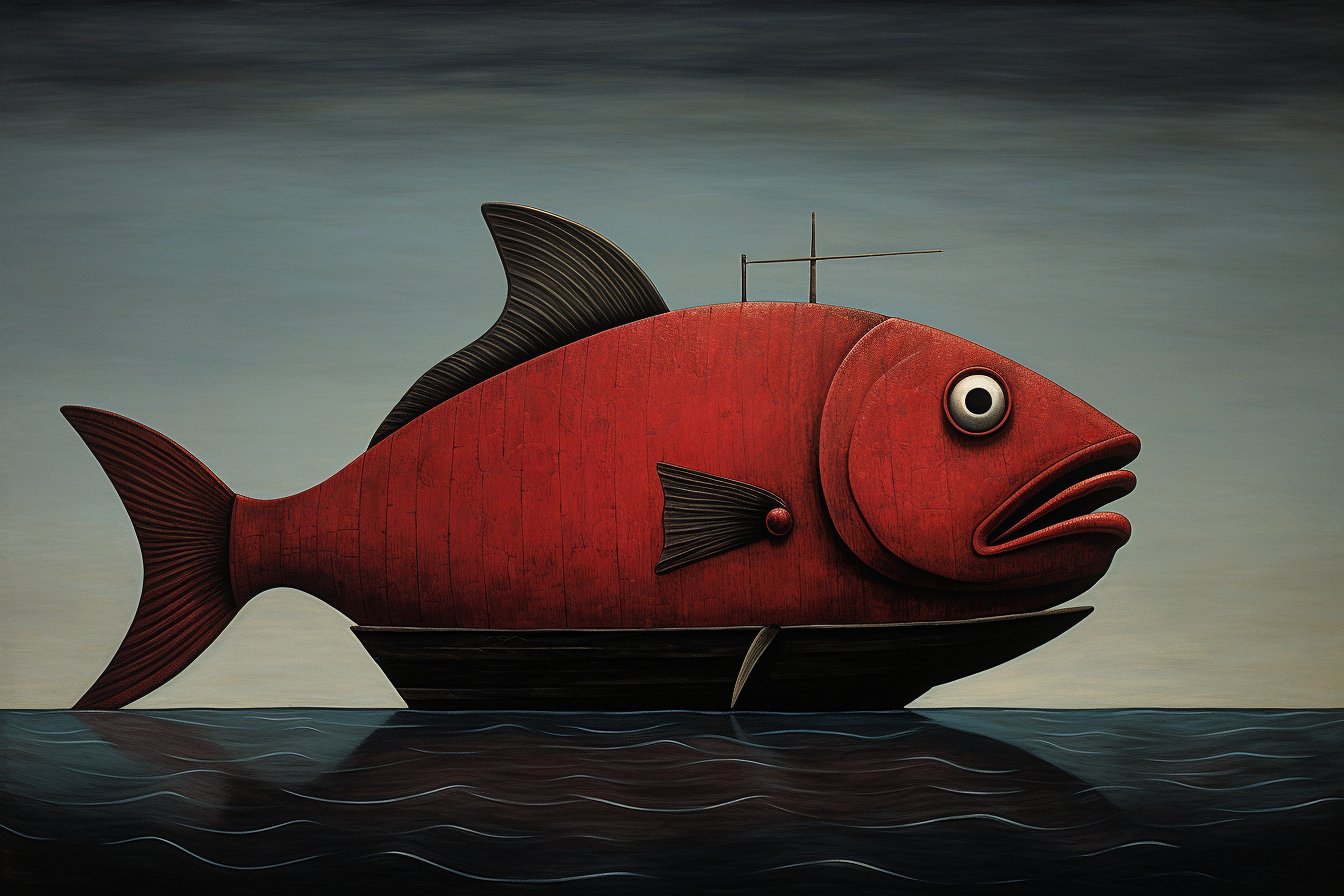This artwork, a richly detailed color illustration, depicts an enormous reddish-brown fish, so large that it dwarfs the small rowboat it rests in. The boat, made of dark wood, appears to be adrift on a dark blue ocean, with white wavy lines indicating gentle ripples. The fish, which spans almost the entire width of the illustration, has a textured appearance suggesting it might be crafted from wood. Its profile shows a slightly open mouth with a red tongue peeking out, and a round white eye with a black pupil staring directly at the viewer, giving it a shocked expression. Black dorsal and side fins accentuate its massive body. Above, the sky transitions from a menacing near-black at the top to lighter shades of blue and beige-gold below, evoking the feel of an impending storm. This striking illustration masterfully blends elements of surrealism and whimsy, creating a captivating visual narrative.